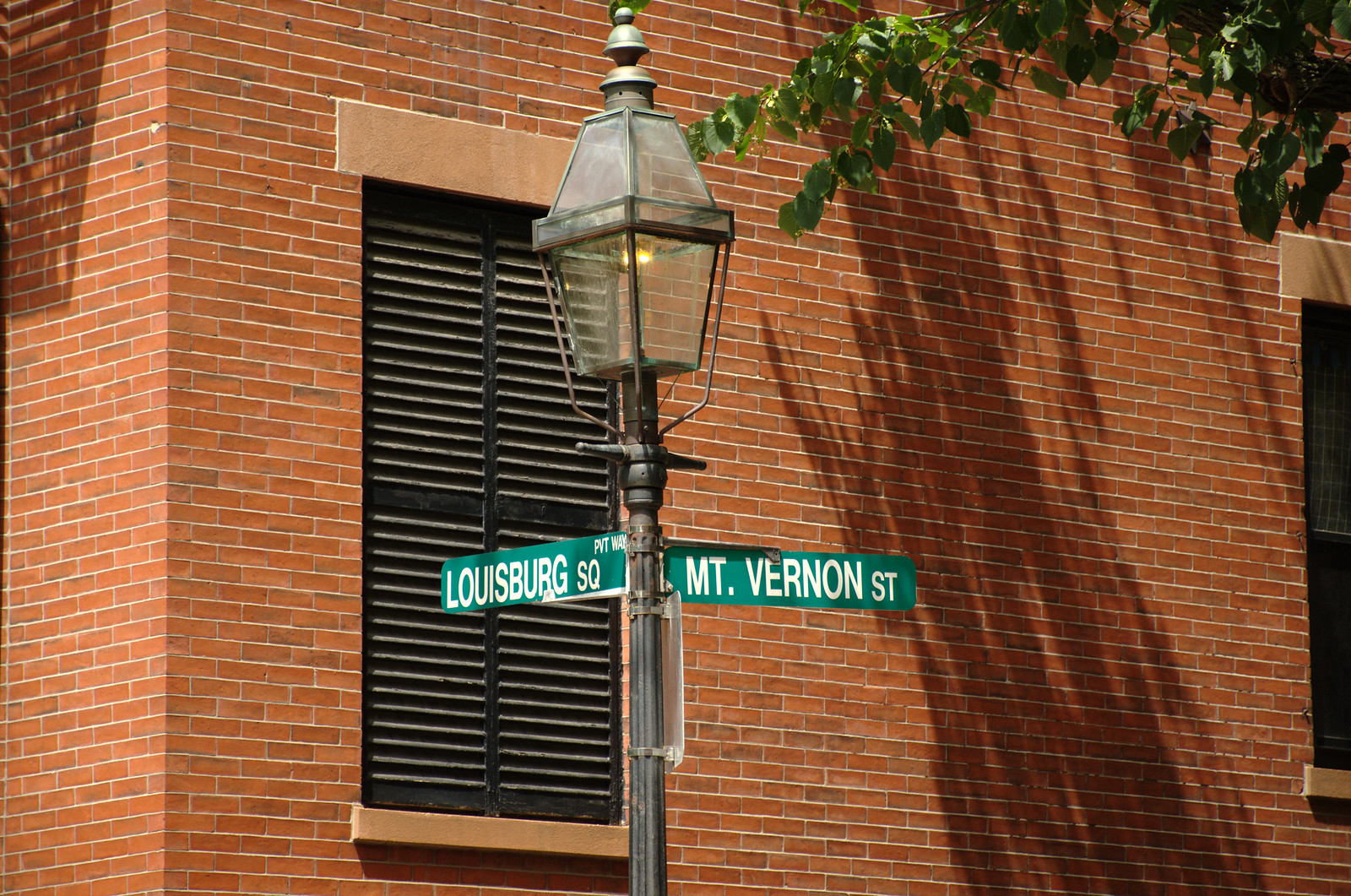This color photograph captures an old-fashioned, antique bronze street lamp with intricate details. The lamp features four trapezoidal faceted glass panels, and it's supported by an ornate post with vertical grooves. The top of the street lamp is adorned with three decorative brass fittings that taper to a rounded brass finial. Attached to the lamp are two green street signs with white text, one reading "Louisburg Square" and the other "Mount Vernon Street."

In the background, a tall red brick building is visible, showcasing neatly stacked bricks, sandy-colored lintel beams, and sills that contrast with the red façade. The building has two windows with black French plantation-style shutters, adding to the historic charm. The scene is set on a sunny day, with shadows from a nearby tree and its green leaves extending into the upper right-hand corner of the photograph.